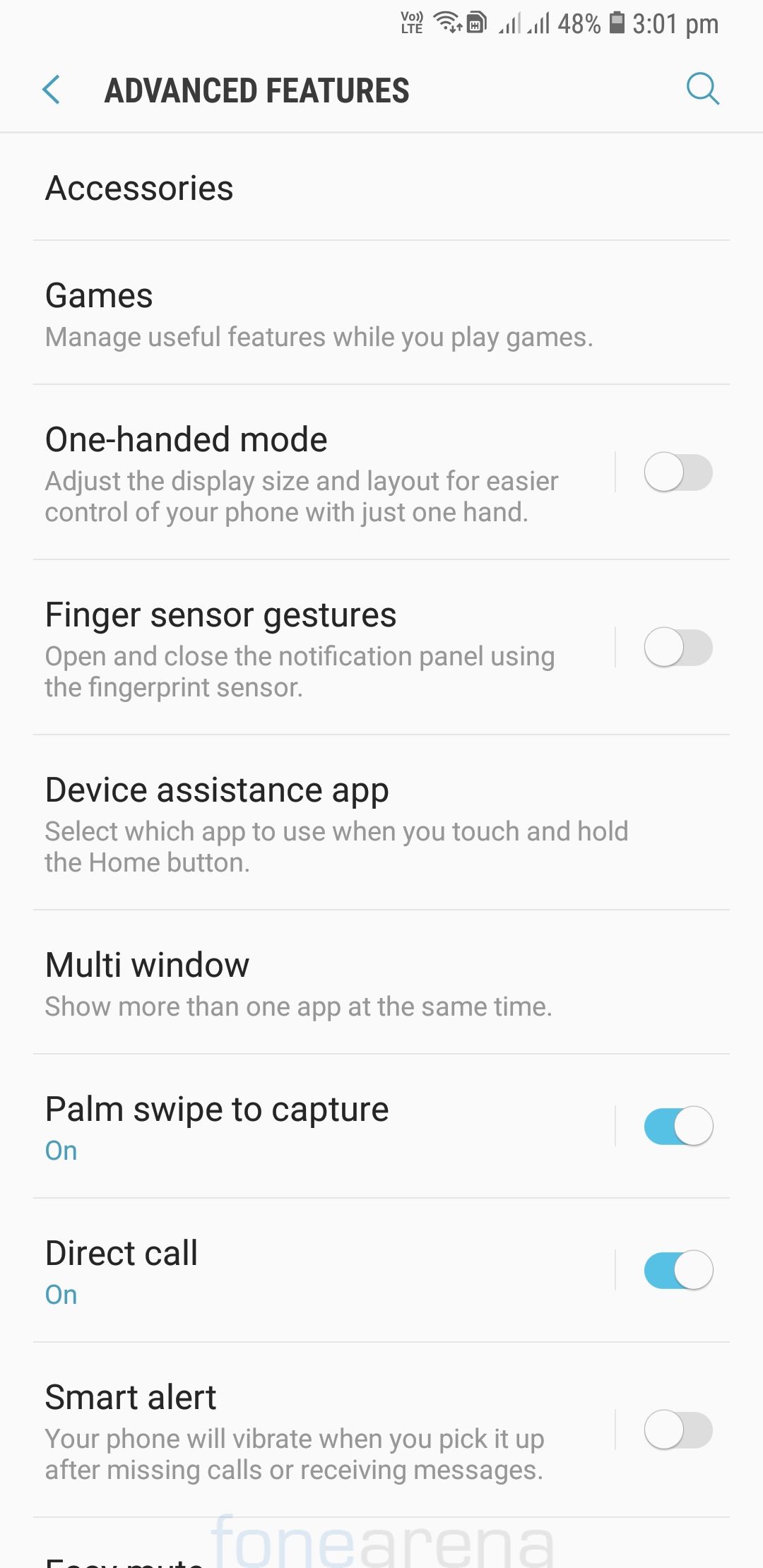A detailed screenshot captured from a smartphone displays a settings menu under the section labeled "Advanced Features" on a clean white background with black text. 

At the top of the screen, black icons indicate the status of Wi-Fi, battery life at 48%, and the current time, displayed as 3:01 PM. Below these icons, a blue back arrow and a blue magnifying glass icon flank the "Advanced Features" heading. The categories within this menu are separated by thin gray lines for clear differentiation.

The first category is "Accessories," followed by "Games," which includes the description: "Manage useful features while you play games." Next is "One-handed mode," allowing the adjustment of display size and layout for easier control of the phone with just one hand; this option is marked by a small gray circle.

Following this is "Finger sensor gestures," which enables opening and closing the notification panel using the fingerprint sensor, also marked by a gray circle. The "Device assistance app" category allows the user to select which app to use when touching and holding the home button. The "Multi-window" option provides the capability to show more than one app at the same time.

Further down, the "Palm swipe to capture" feature is turned on, indicated by a white circle pulled over on a blue bar. Similarly, "Direct calls" is also enabled, with an "On" label in blue and the corresponding white circle on the blue bar. Lastly, "Smart alerts" is described as a feature making the phone vibrate when picked up after missing calls or receiving messages, and it is followed by a white circle.

At the bottom of the screenshot, a watermark from "PhoneArena" (stylized as "fonEarena") is visible, along with some partially cut-off black text. The image is clear with large, easy-to-read font and no other objects of note present.